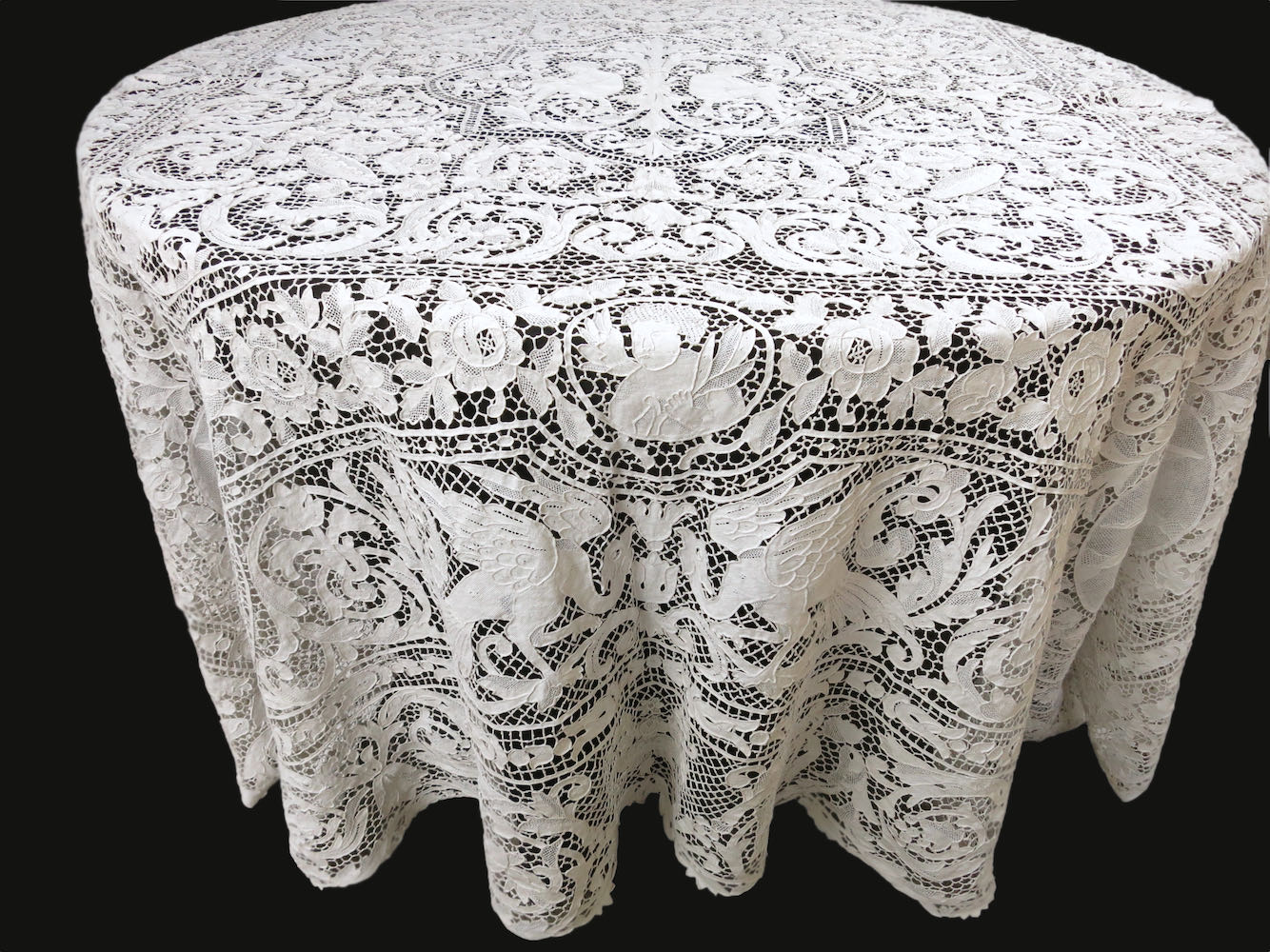The image features a round table draped with an intricate white lace tablecloth, set against a completely black background which accentuates the tablecloth's detailed design. The lace showcases a variety of floral patterns, including roses, as well as mythical and angelic figures like cherubs with wings, a person holding leaves or olive branches, and creatures resembling winged lions with human faces. The tablecloth also features phoenix-like birds within the lacework. This ornate tablecloth covers the entire table and reaches down to the floor, suggesting it could be used for a special occasion or setting, such as in a kitchen or potentially at a wedding or other formal event. There is no text visible in the image. The overall effect is one of elegance and meticulous craftsmanship.